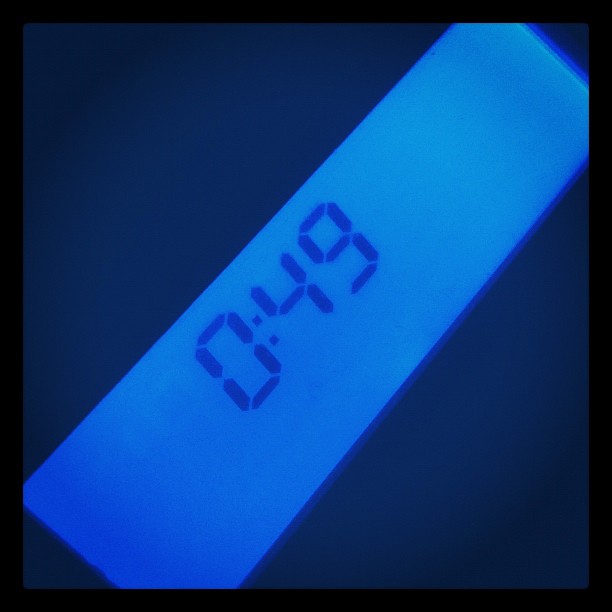This close-up photograph captures a digital timer, prominently displaying "0:49" on its screen, likely indicating 49 seconds remaining. The setting is extremely dark, enhancing the high contrast of the backlit LCD display against its surroundings. The timer's screen has an aquatic blue background with dark blue or black numbers. The image is oriented diagonally, running from the bottom left to the top right, and framed by a black border. The stark simplicity and the high contrast of the illuminated timer make it the sole focus of the photo, reminiscent of an isolated digital device in a dark environment, possibly underwater or at night.